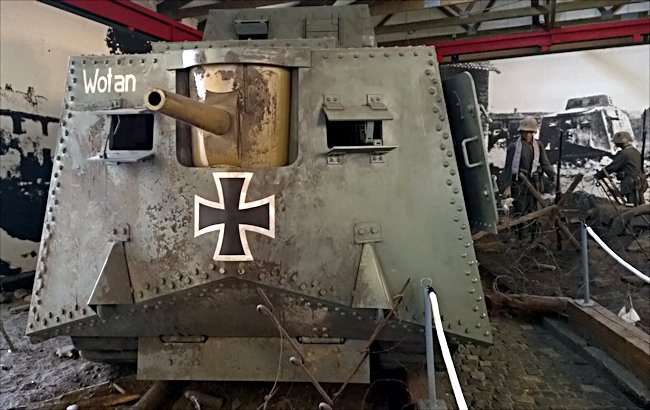The photograph captures an exhibit within a war museum, prominently showcasing a World War I German Panzer tank, identified by the inscription "WOTAN" painted in white on the top left corner. The tank, displaying the emblematic black cross with a white outline, is set amidst a realistic wartime diorama. It features a copper-colored gun barrel protruding from its center, flanked by two lookout holes giving it a visage reminiscent of a knight’s faceplate. The groundwork beneath the tank includes stone steps and areas covered with dirt, while wooden X-shaped barricades and barbed wire recreate a battlefield atmosphere. Surrounding the tank, large photographs depicting World War I scenes enhance the historical ambiance, and mannequins dressed in period-appropriate military attire add a lifelike touch to the display. The exhibit is further framed by big red steel bars overhead, contributing to the detailed and immersive presentation of this museum artifact.